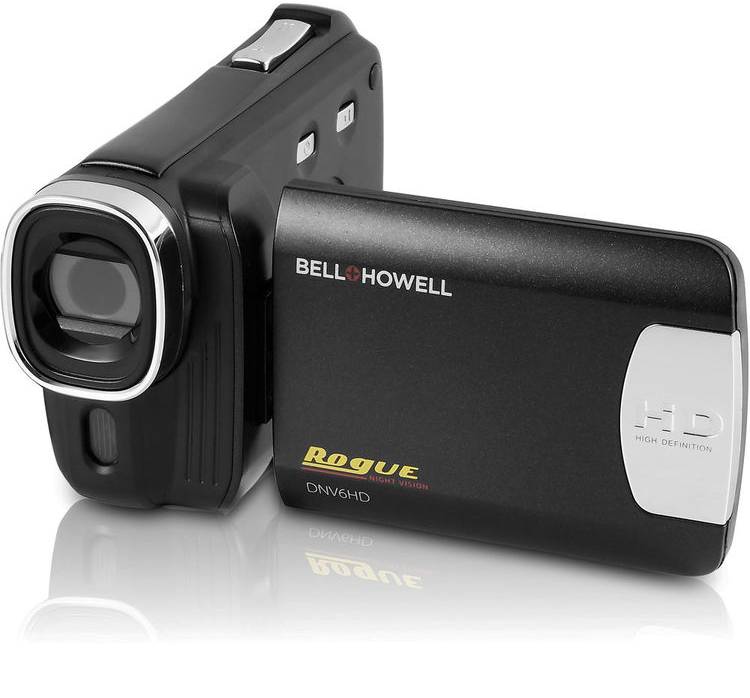This is a high-definition handheld camcorder by Bell & Howell, model number DNV-6HD, featured in a promotional photo. The camcorder, predominantly black with silver detailing around the lens, is slightly larger than hand-size and has a sleek, rectangular shape with rounded edges. The camera is shown with its flip-out screen extended, which is common for viewing while filming. The flap on the screen features several logos and labels: "Bell & Howell" in white font, "ROGUE" in a retro yellow font with an extended 'G' beneath "NIGHT VISION" in red, and "HD High Definition" in metallic lettering. The reflective surface beneath the camcorder highlights its glossy finish, casting a faint shadow. This vintage-styled model appears brand new, sitting on a bright white, seamless background.